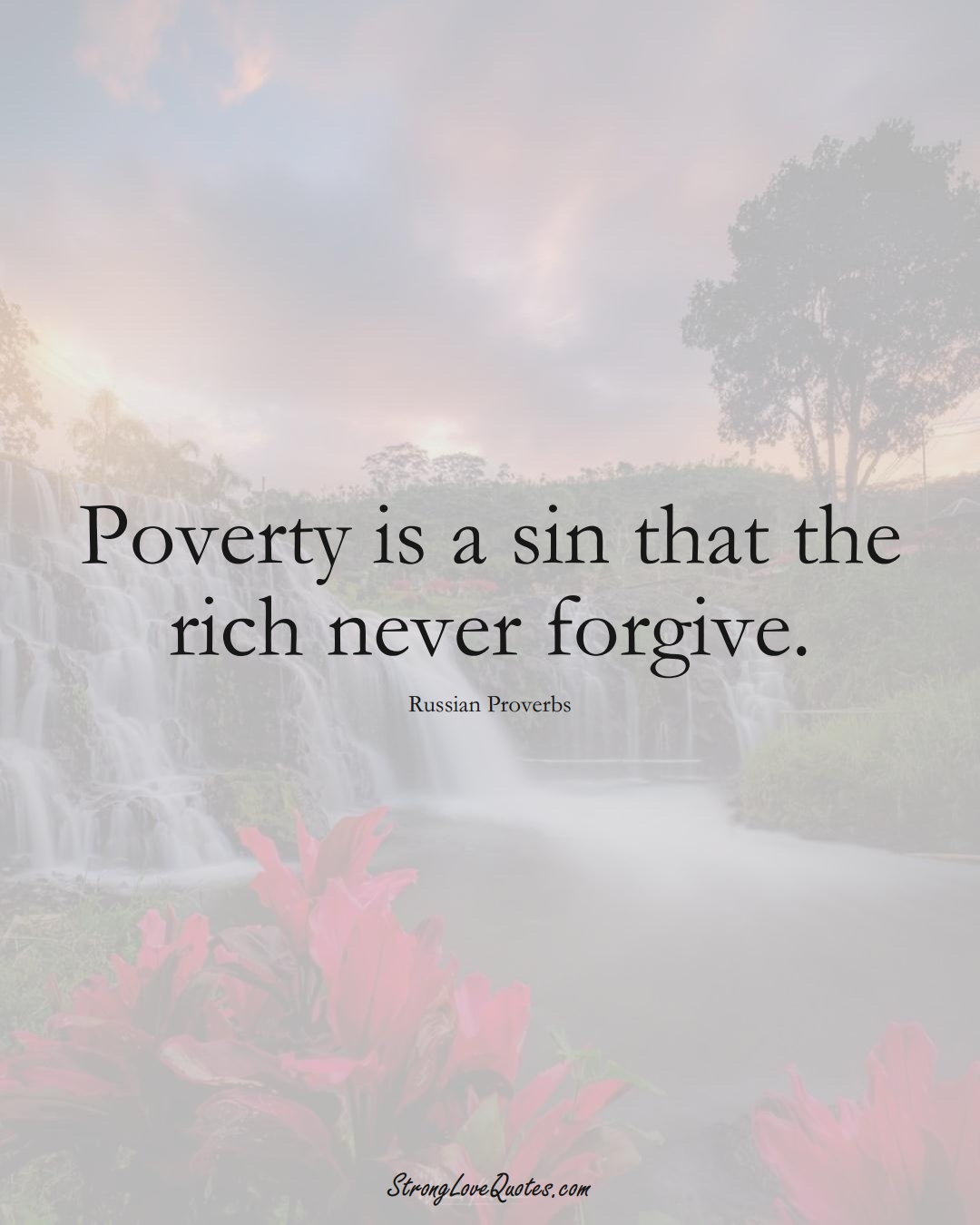The image displays a quilt picture with an emphasis on its inscriptions, set against a picturesque background. The backdrop features a serene landscape with a majestic waterfall cascading down the left side into a tranquil pool surrounded by lush greenery. To the right, rolling hills and trees are visible under a captivating, multicolored sky that could be either sunrise or sunset, enhanced by hues of orange, blue, pink, and off-white. Prominently displayed at the top of the image in bold black letters is the quote, "Poverty is a sin that the rich never forgive." Beneath this, in smaller black font, it reads, "Russian Proverbs." At the bottom center, in cursive black letters, is the text "StrongLoveQuotes.com." The overall composition, with its striking natural elements and poignant message, evokes a meme style intended for online sharing.